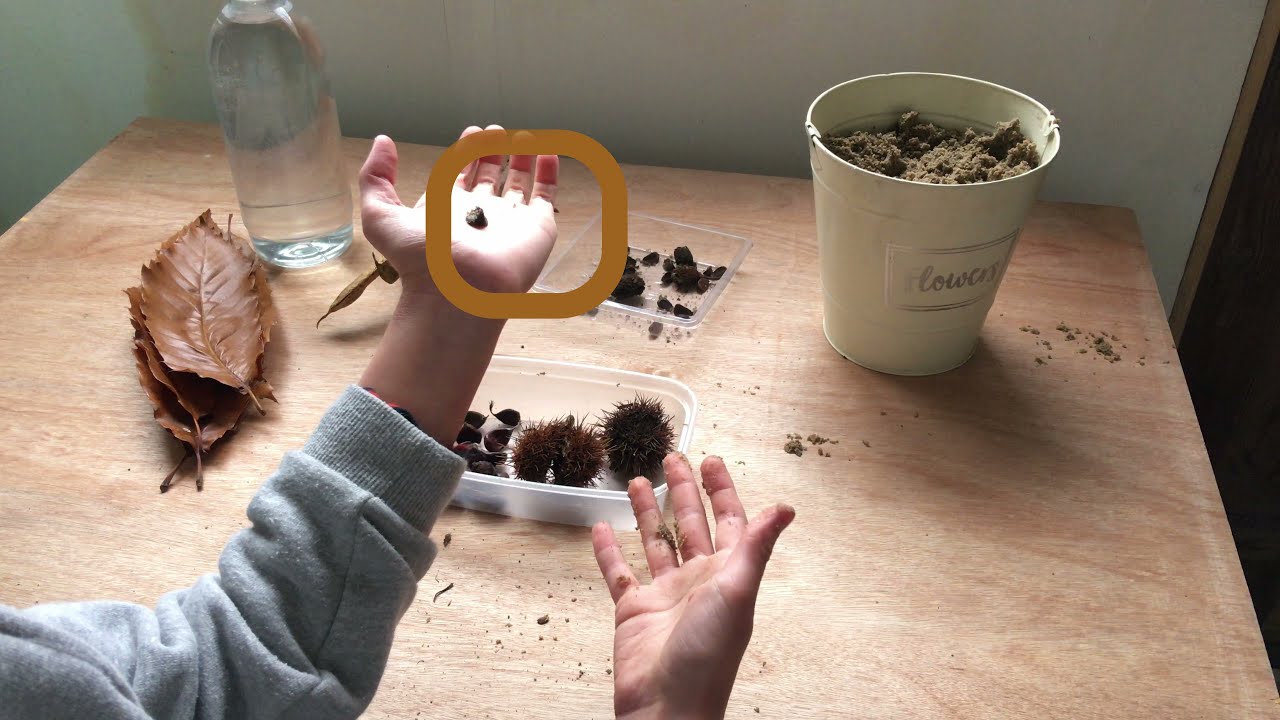This horizontal rectangular image captures a child's hands engaged in an earthy activity, possibly a science or earth project. The child, wearing a gray sweatshirt, holds a small, brown object in the palm of their left hand while extending their right hand, which is speckled with dirt or grass. Both hands are positioned above a clear rectangular tray filled with larger, pointed, brown circular objects. The background features a light brown wooden table occupying most of the frame, against a stark white wall. On the left side of the table, there is an empty glass bottle next to a stack of brown leaves. Toward the back right of the table sits a white cup adorned with printed flowers and filled with dirt. Additionally, a white metal container labeled "flowers" containing dirt and various earthy items such as dry leaves and pine cones are scattered across the table, adding to the scene's intricate, naturalistic details. A mustard-yellow rounded-edge square highlights the brown object in the child's left hand, drawing attention to the focal point of the image.